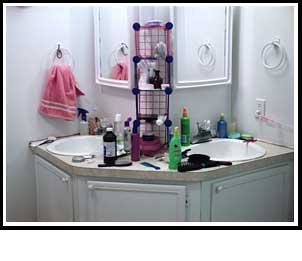The image captures a unique corner bathroom setup featuring a double vanity sink arrangement. Each sink is positioned at a 90-degree angle from one another, with a middle section forming a 45-degree angle. Behind each sink is a mirror, placed at a 90-degree angle to its counterpart. Each sink is equipped with a towel ring: the left towel ring holds a pink rose-colored towel with a stripe, which is reflected in the mirror. The vanity surfaces are cluttered with various products, including hairbrushes, combs, a brown bottle with a white label, and several green bottles with yellow or golden tops. A dark blue bottle with a yellow or golden top is also visible. To the right of the rightmost sink, there is an electric outlet. The vanity includes cabinet doors beneath all three surfaces, providing storage space in this corner-oriented double sink design.